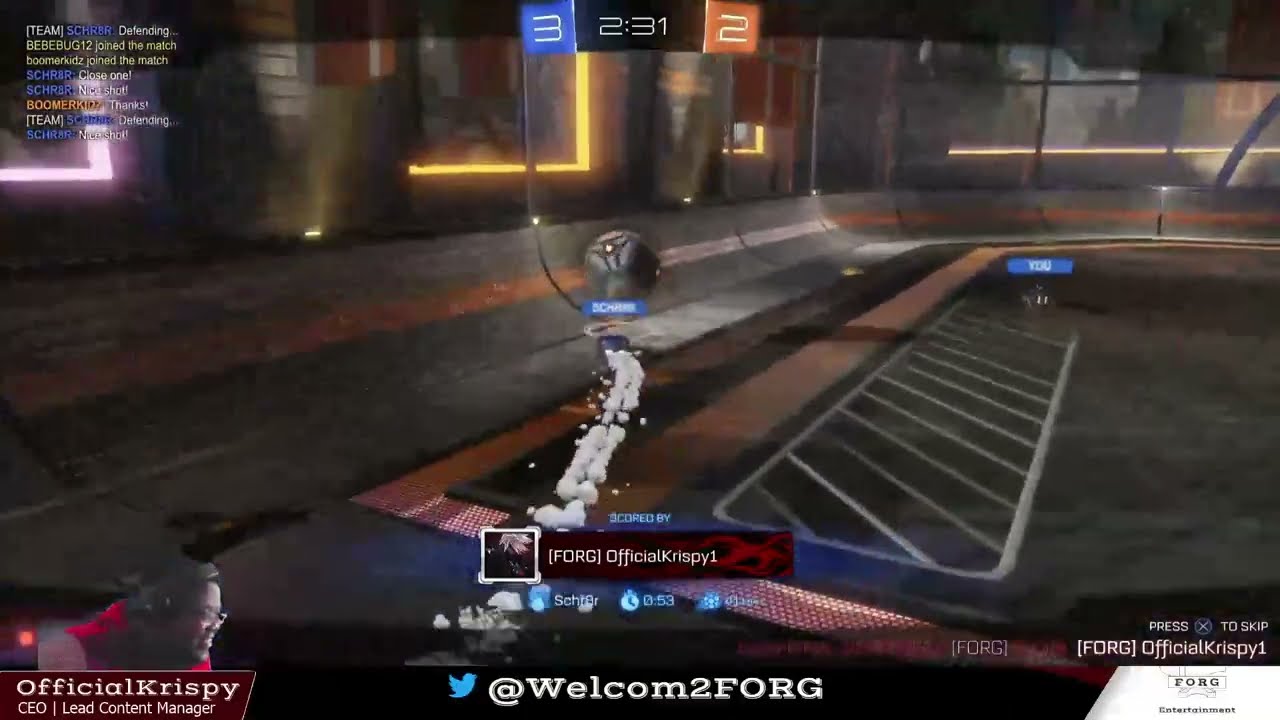The screenshot showcases a Rocket League game with a gray-colored field and an orange-striped ramp wall on the left. In the center-right, a white triangle with diagonal lines and a white character with "YOU" highlighted in blue is visible. A string of white balls connects to this character, leading upwards to the top of the screen. 

At the top center, game stats are displayed: a blue square with the number "3" on the left, a translucent section with "2:31" in the middle, and an orange square with the number "2" on the right. In the lower-left corner, a picture of a black male streamer wearing glasses and black headphones is shown. Beside this avatar, there's white text reading "Official Krispy 1" and "CEO Lead Content Manager." 

Below this, scores and a Twitter symbol are displayed, with the text "@ WEL COM T F.O.R.G" visible. In the bottom right, more white text reads "PRESS X TO SKIP," and underneath, it says "F.O.R.G. Official Krispy 1" and further below, "F.O.R.G. Entertainment." The upper left corner contains text that says "Team Defending" in white, with additional dark blue, orange, and yellow texts that are partly unreadable.